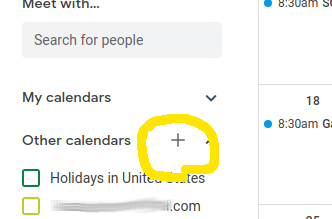This is a cropped screenshot of a calendar application, focusing on a few specific elements. The image is very small and square, with most of the content cropped out. 

In the top left corner, the bold, dark gray text "Meet with…" is partially visible and followed by ellipses, indicating truncated content. Below this is a search box containing the placeholder text "Search for people" in gray letters.

Directly beneath the search box, there's a section titled "My Calendars." This is printed in bold and located at the top left of the section, accompanied by a dropdown arrow on the right.

Further down, the left side of the image displays the "Other Calendars" section with the title aligned to the left. To its right, there is a plus sign, which has been emphasized by a yellow circle overlaid onto the screenshot. This highlight appears to serve as an instructional or navigational aid.

On the right-hand side of the screenshot, a portion of the calendar grid is visible, albeit cropped. The top entry features a blue dot next to the time "8:30 a.m." and the letter "S," suggesting the start of an event. Further down, another entry indicates the day as "18th," also marked by a blue dot next to "8:30 a.m." This repeated time suggests recurring or multiple events scheduled at the same time.